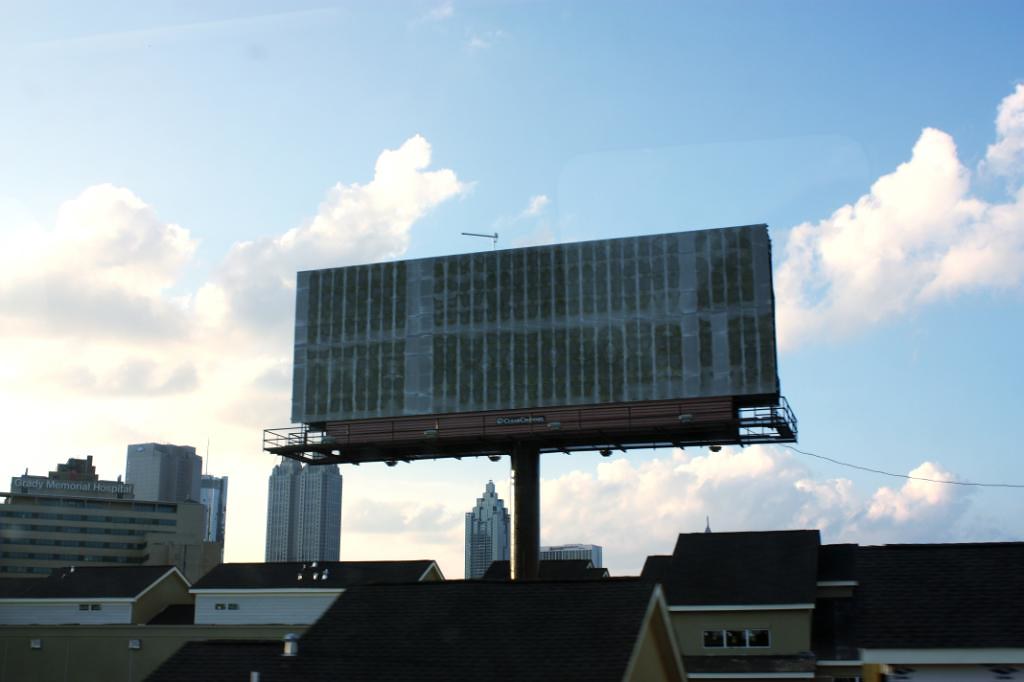This image is of a large blank billboard situated in a downtown area, captured with an older digital camera. The billboard, which is faded dark green and gray in vertical patches, dominates the center of the photo and has some scaffolding on it. The photo includes the rooftops of various buildings in the foreground, primarily two-story townhouses in hues of light blue, light brown, and black. The backdrop showcases a few high-rises and taller buildings further in the distance. The sky is a light to medium blue with scattered fluffy white cumulus clouds, and sunlight is streaming from the left, indicating it is late afternoon.